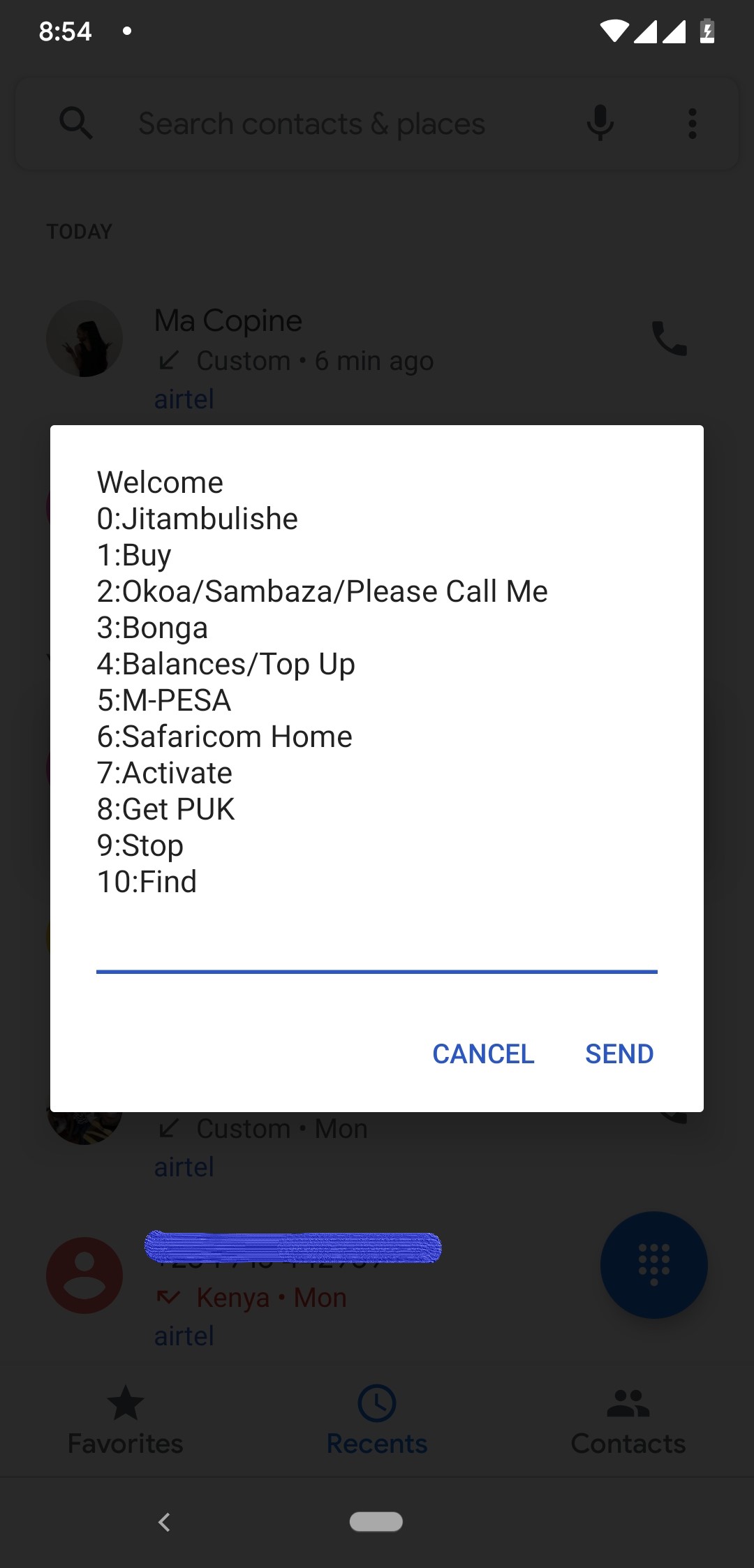This is a screenshot captured from a cell phone. The screen has a solid black background. In the upper left corner, the time is displayed in white text as '8:54'. To the right of the time, a symbol indicates that Wi-Fi is enabled.

Centrally positioned within this black background is a large white rectangle featuring text in black and blue. At the top of this rectangle, the word "Welcome" is prominently displayed. Below "Welcome," there is a numbered list consisting of:

1. **JIT AM BLEACH 1:5**
2. **ACOA/SAMBASA/Please Call Me**
3. **BANGA**
4. **Balances/Top Up**
5. **M PESA**
6. **Safari Calm Home**
7. **Activate**
8. **Get Puck**
9. **Stop**
10. **Find**

Underneath this list, a thin horizontal blue line separates the text from the bottom section of the white rectangle. In the lower right corner of the white box, there are two options: "Cancel" and "Send".